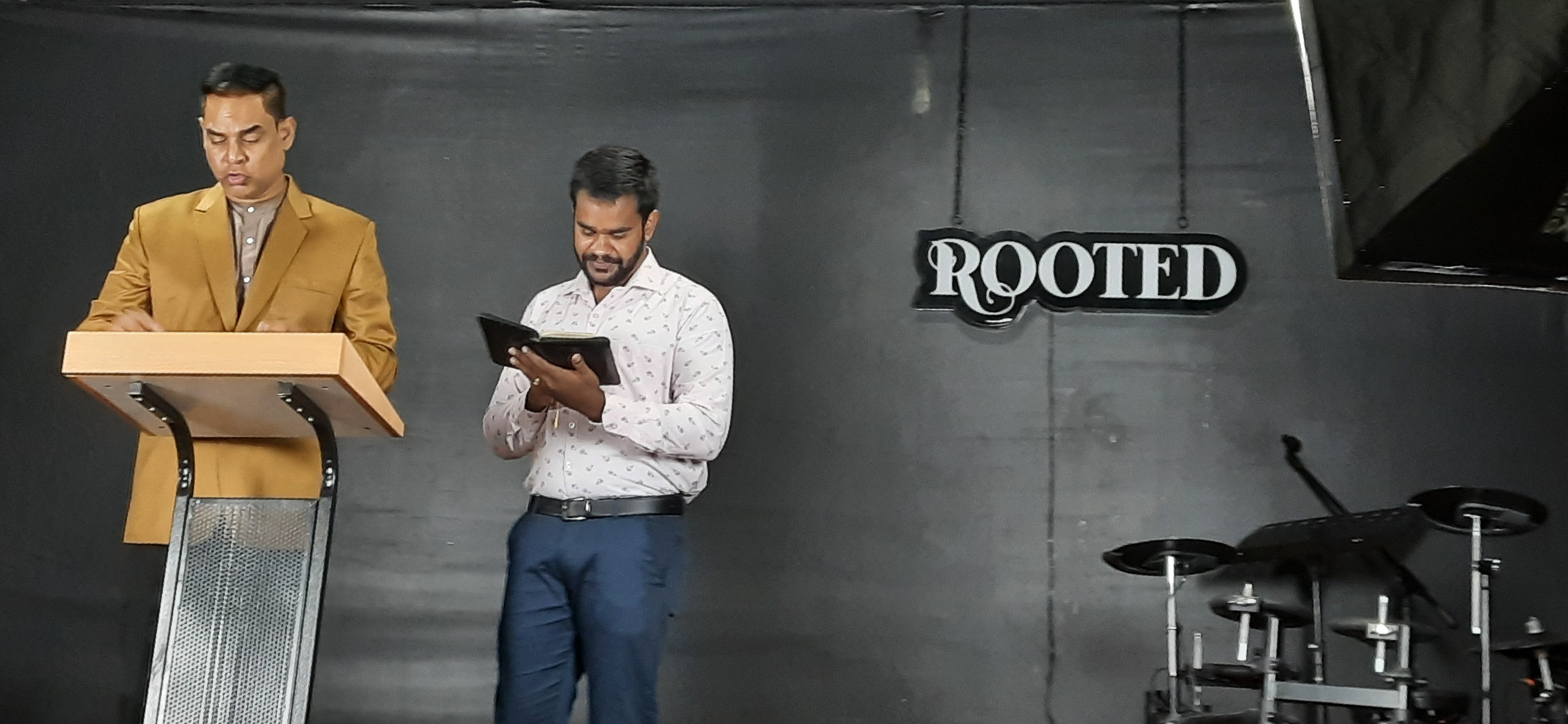The image depicts an indoor scene with two Indian men. The man on the left stands at a wooden podium with a metal base, featuring decorative black curvy elements. He is dressed in a tannish brown sports jacket over a tan shirt with buttons, and has short black hair. He appears to be speaking. To the right, a slightly smaller man with black hair is wearing a white-collared shirt, blue pants, and a black belt. He is holding an open black book and seems to be reading or looking through it. The background wall is gray and prominently displays the word "ROOTED" in white, all capital letters with a black outline. In the bottom right corner of the image, there appears to be a drum set or similar metal, round objects, indicating the presence of musical instruments. Overall, the setting is dimly lit with a plain, unadorned backdrop, focusing attention on the two men and their activities.